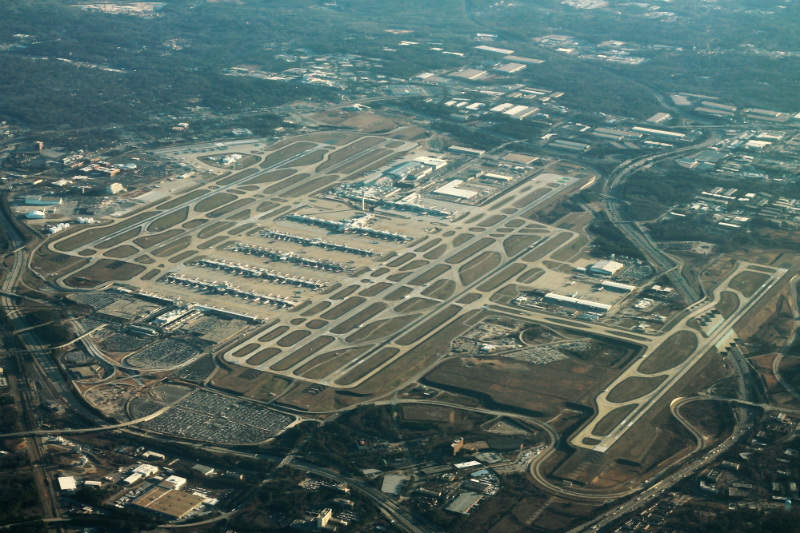This aerial photograph, likely taken from an airplane or drone, presents a wide-angle view of a large industrial complex that possibly resembles a factory or an old airport. Dominating the center of the image is a substantial building with adjacent warehouses, surrounded by a notable number of parked cars lined up in neat rows. The scene is characterized by an extensive network of roads and highways that seem to loop and intertwine around and through the industrial area, providing clear connectivity. In the upper left, a dense cluster of trees contrasts with the industrial landscape, while the peripheral areas show scattered houses and various smaller buildings, suggesting a mix of residential and industrial zones. The photograph, appearing somewhat faded and washed out in green hues, hints at either age or poor lighting conditions, enhancing the feel of an older yet detailed snapshot taken during the daytime.